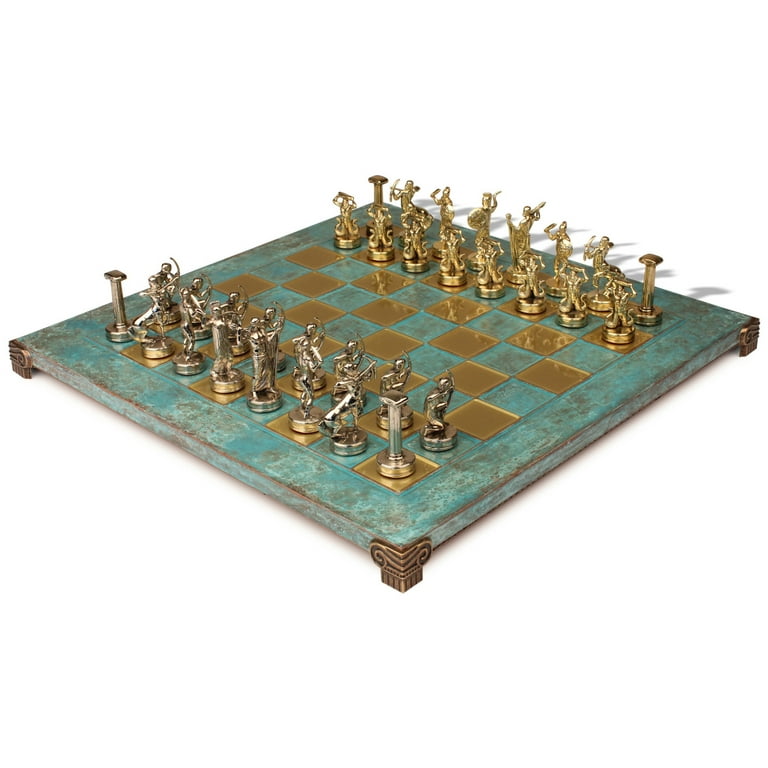The image showcases a luxurious and highly detailed chess set against an all-white background. The chessboard itself is primarily a turquoise or green alabaster stone, embellished with reflective gold glass tiles that form alternating squares. The board is supported by short, fluted brass legs at each corner, giving it the appearance of floating on a white surface. Positioned at an angle with one corner facing the bottom center of the image, the chess pieces are meticulously crafted and resemble tall, slender warriors. The yellow brass pieces are situated at the back of the board, while the silver nickel pieces occupy the front. The ornate chess pieces include figures with bows and swords, with taller kings and queens, and distinctive rooks and pawns. The overall style of the photograph is realistic, capturing the intricate details and opulence of this unique chess set.